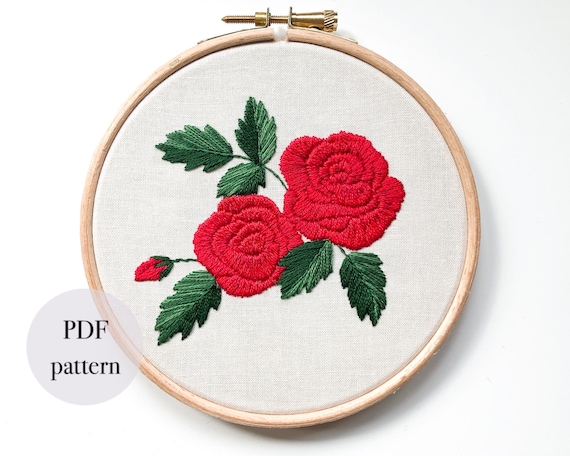This full-color vertically rectangular photograph, subtly enhanced, features a delicate needlepoint design. The background is an almost imperceptible off-white, lending a clean and simple canvas for the artwork at its center. Dominating the scene is a white cloth secured within a light brown embroidery hoop, which itself is tightened with a golden screw to ensure tautness.

Central to the image are three beautifully stitched roses — two in full bloom and one still budding — rendered in vibrant red thread. Surrounding the roses are six meticulously embroidered green leaves, each with pointed edges and intricate detailing that adds to the lifelike quality of the needlework. The image captures the fine texture of the cloth and the precision of the stitching.

In the lower left corner, a translucent off-white circle bears the black text "PDF pattern," subtly indicating that this intricate design is available as a pattern for enthusiasts. The composition, rich in color and detail, evokes the warmth and dedication of traditional craftwork, elevated by minor digital enhancements that bring out the vibrancy of the stitches.